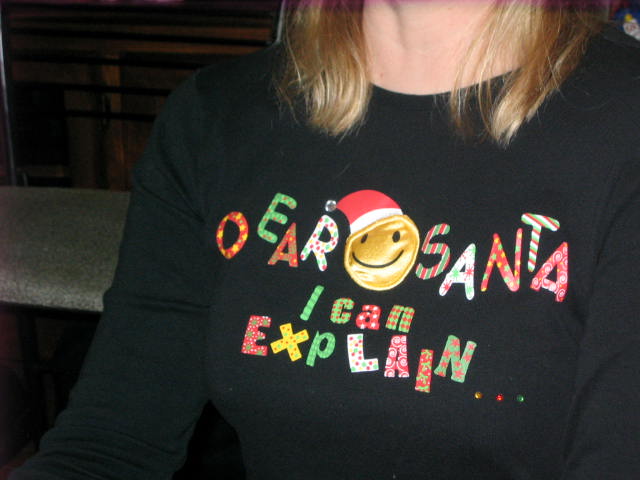A close-up photograph captures the chest area of a woman wearing a long-sleeve black shirt. Portions of her hair and neck are visible, but her face and waist are out of the frame. The shirt features a playful and colorful design with the word "DEAR" prominently sewn in various materials. Next to the letters, there is a cheerful yellow smiley face adorned with a Santa hat. Below this, the phrase "Santa, I can't explain..." appears, punctuated by three dots. The design uses a vibrant mix of green and red colors, contributing to the shirt's humorous holiday theme.